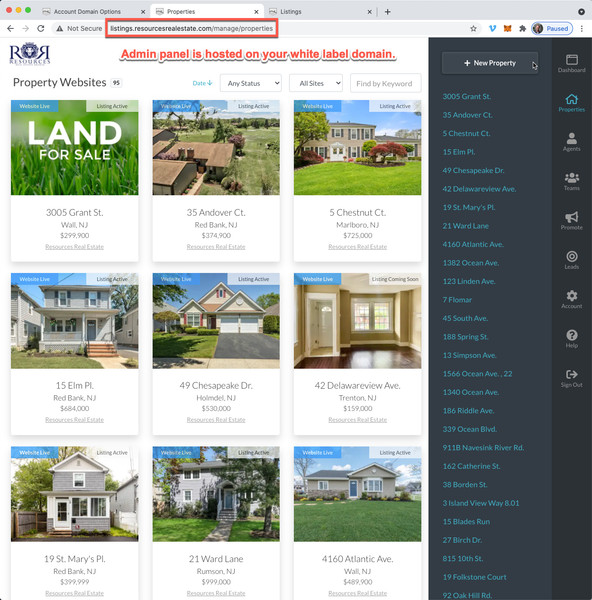The image is a screenshot from a real estate listing website featuring both the logo "R&R Resources" and its tagline, "Admin panel is hosted on your white label domain." The listings include various properties for sale, each depicted with an image and detailed information. 

On the left, there is a plot of land with lush green grass, located at 3005 Grant Street, Weill, New Jersey, listed for $299,900. Adjacent to this is a house for sale at 35 Andover Court, Red Bank, New Jersey, priced at $374,900. Further to the right, a luxurious mansion at 5 Chestnut Court, Marlboro, New Jersey, is available for $725,000.

Below the mansion is a two-story house located at 15 Elm Place, Red Bank, New Jersey, with a price tag of $684,000. To the right of this listing is another home for sale at 49 Chesapeake Drive, priced at $530,000. Each property listing is accompanied by relevant imagery and clear, detailed information on the location and price.